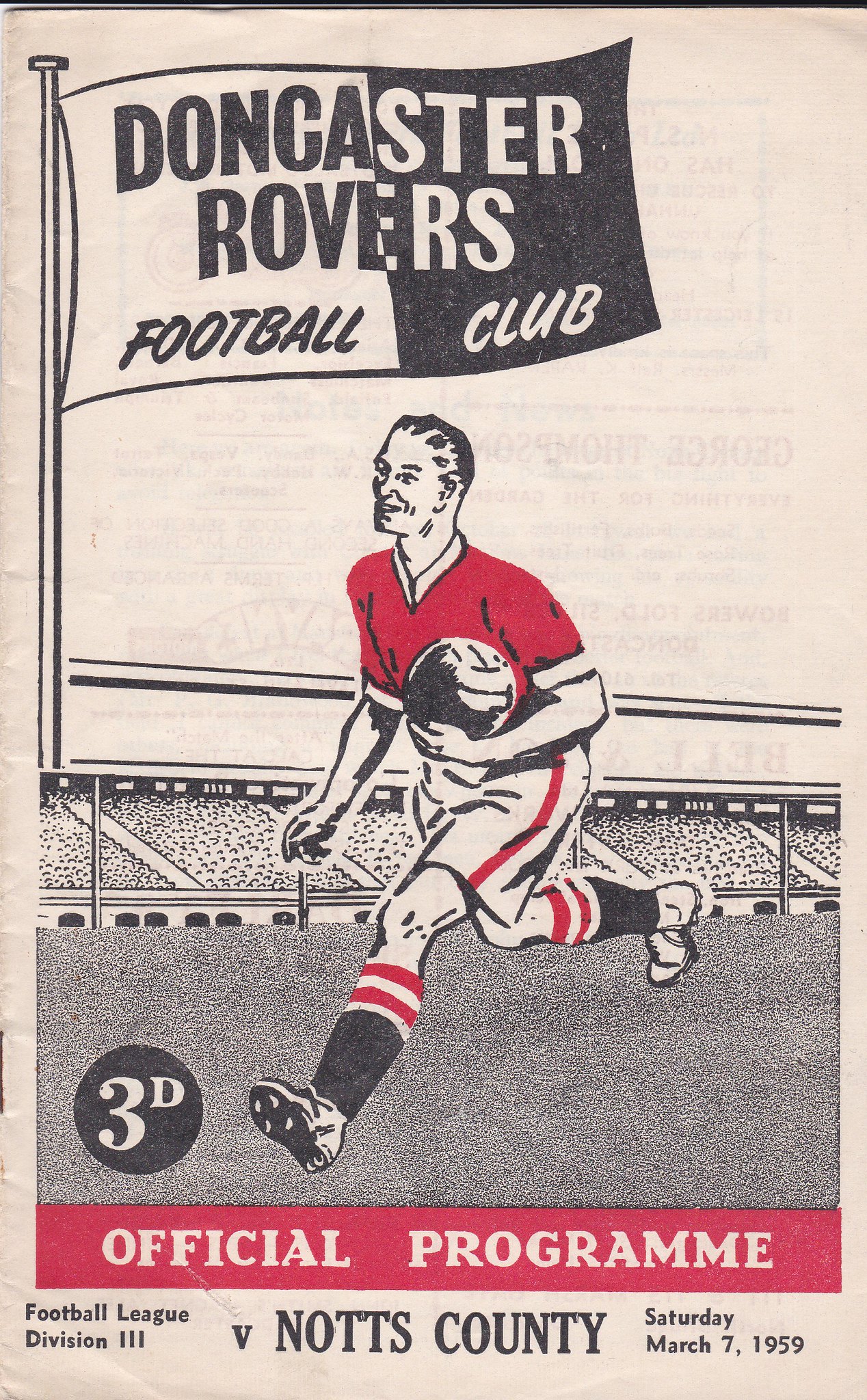The cover of the program is printed on white paper that has darkened with age to a tan hue, giving it a vintage look. At the top of the cover, there's a stylized cartoon flag split into white and black halves, which reads "Doncaster Rovers Football Club." Below the flag is a detailed hand-drawn illustration of a man in a red jersey and white shorts with a red stripe. He is holding a soccer ball and running on a soccer field, depicted with stands full of spectators in the background. The man is also wearing black socks with red and white stripes at the top and white soccer cleats. Next to the man, there's a black circle with the text "3D" in white font. Beneath the illustration, a red banner reads "Official Program," followed by "Football League Division Three v Notts County" and the date "Saturday, March 7th, 1959." The paper shows signs of wear, including distress marks, wrinkles, and rusted staples along the left-hand side, indicating its age and authenticity.